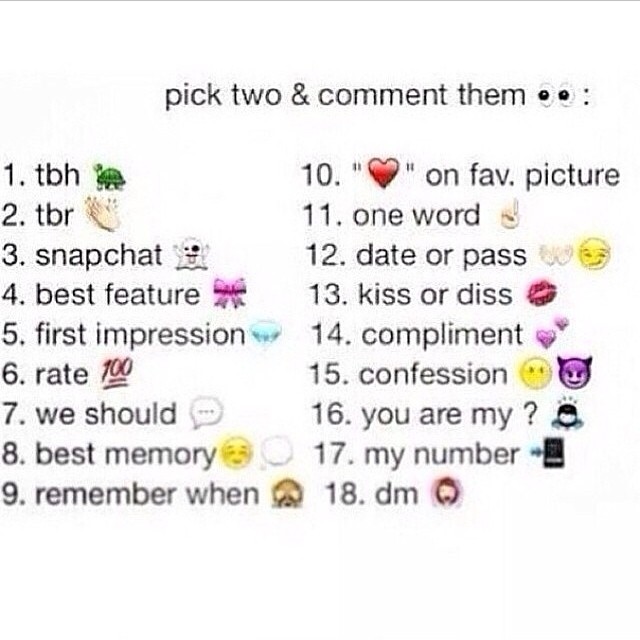The image features a social media meme in landscape orientation, combining graphic design and typography with emojis. A thin pinstripe border runs horizontally at the top. Just below, in black print, the headline reads "Pick two and comment them" alongside two black-and-white eyeball emojis looking left. Following the headline, there are two columns numbering 1 through 18, each item paired with an emoji. The left column lists: 1. TBH (green turtle), 2. TBR (clapping hands), 3. Snapchat (ghost), 4. Best Feature (pink bow), 5. First Impression (blue diamond), 6. Rate (red 100 with double underlines), 7. We Should (white speech bubble with ellipses), 8. Best Memory (blushing emoji and white puffy cloud), and 9. Remember When (monkey covering eyes). The right column continues with: 10. Heart on Fav Picture (red heart), 11. One Word (index finger pointing up), 12. Date or Pass (two hands out and a smirking face), 13. Kiss or Diss (red lips), 14. Compliment (two purple hearts), 15. Confession (emoji with no mouth and purple devil emoji), 16. You Are My Question Mark (exasperated person icon), 17. My Number (black telephone), and 18. DM (woman’s face). The overall design suggests it may be a screenshot from a cell phone, inviting social media interaction by asking viewers to choose and comment on two options from the list.